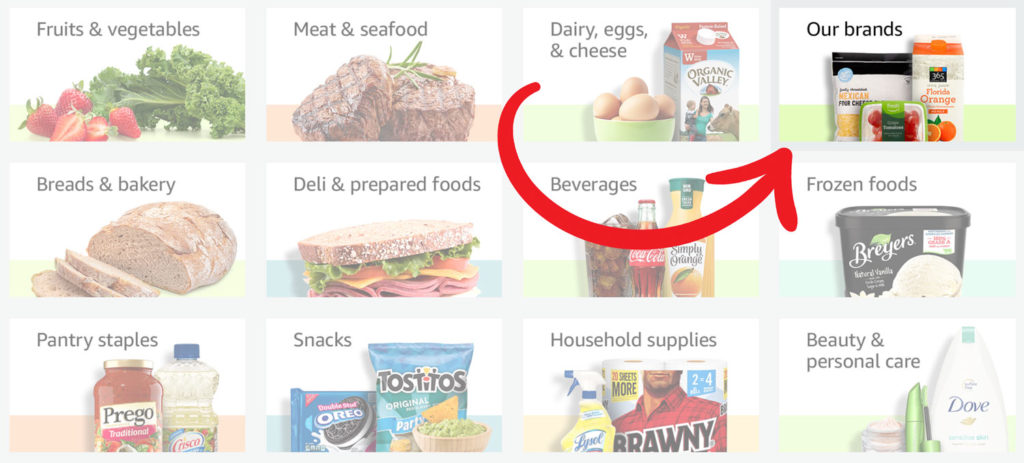This image shows a detailed menu of a grocery store's online food selection website. The menu is compartmentalized into various categories with corresponding visuals. 

- **Fruits and Vegetables:** Depicts fresh cherries and lush kale.
- **Meat and Seafood:** Displays two round steaks, showcasing fresh meat options.
- **Dairy, Eggs, and Cheese:** Features organic products, including a carton of eggs and Organic Valley milk.
- **Our Brands:** Highlights the store brand products with a red arrow pointing to this section for easy identification.
- **Breads and Bakery:** Shows a neatly sliced loaf of bread.
- **Deli and Prepared Foods:** Presents a delicious ham and turkey sandwich with tomato, lettuce, and cheese.
- **Beverages:** Includes a classic bottle of Coca-Cola, a glass filled with iced Coca-Cola, and a glass of orange juice.
- **Frozen Foods:** Features a tub of black vanilla-flavored Breyers ice cream.
- **Pantry Staples:** Shows essential items like Prego pasta sauce and Crisco shortening.
- **Snacks:** Displays popular snacks such as Oreos, Tostitos, and an unidentifiable green snack item.
- **Household Supplies:** Highlights Brawny paper towels and Lysol cleaning products.
- **Beauty and Personal Care:** Showcases Dove lipstick and facial pads.

For more detailed information and to explore further, visit [www.FEMA.gov](http://www.fema.gov).